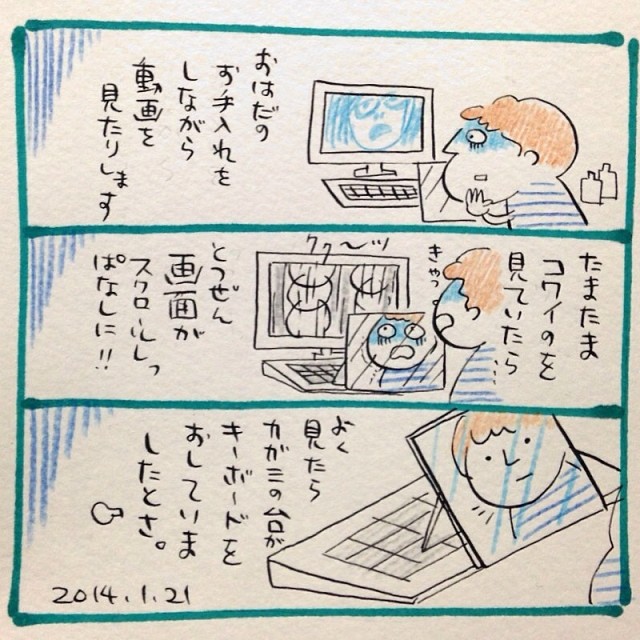This is a hand-drawn and colored cartoon triptych comic strip on a white background with a teal-green border. The comic, dated 2014-1-21 in the bottom left corner, features three horizontal panels. Each panel is flanked by writing in Japanese or Chinese characters. 

In the first panel, a red-haired boy sits in front of a desktop computer, intently staring at the monitor, which displays an image of someone. The second panel shifts to the boy looking at his reflection in a mirror, while still seated at the computer. The third panel offers a closer view, focusing solely on the boy’s face and the mirror, omitting the computer screen entirely. Throughout the strip, the boy's expressions and interactions with the screen and mirror reflect a contemplative mood, enhancing the detailed narrative of the artwork.